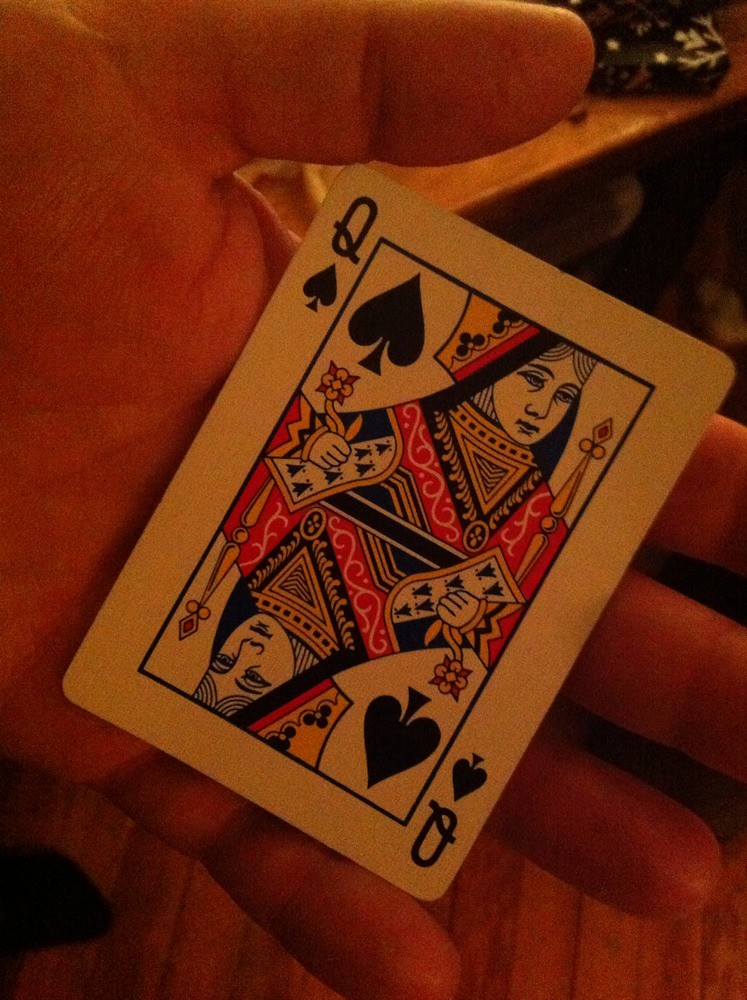In this image, a Queen of Spades playing card is prominently displayed as the main focal point. The classic card, featuring the typical regal depiction of a queen, is held delicately in the left hand of an unseen individual. The hand is open and outstretched, with the card resting against the fingers and the upper part of the palm. The thumb is positioned at the top of the frame while the fingers point downwards and to the right. 

The background hints at a cozy, perhaps intimate setting. Dim lighting casts an orange-red tint over the scene, suggesting a warm atmosphere. Out-of-focus tables and a wooden floor are faintly visible, implying that the photograph was taken in a bar or a domestic space. The overall composition and warm lighting evoke a sense of casual intimacy, capturing a fleeting moment in what appears to be a low-lit, welcoming environment.